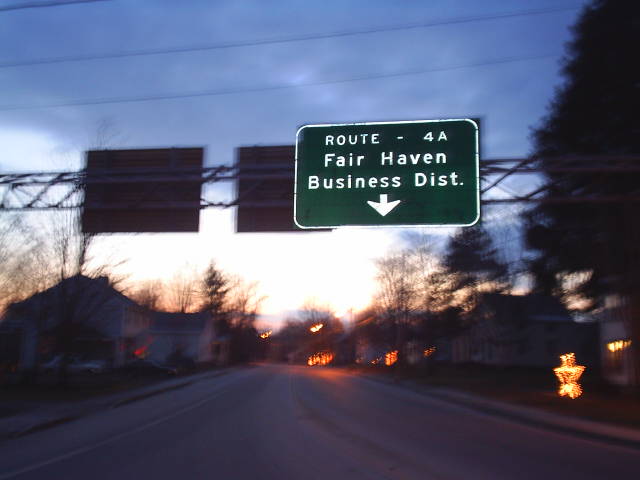This photograph captures a wide, out-of-focus perspective of a road in America, likely Route 4A, based on the visible signage. The road lacks central markings, lined instead with large, detached houses on either side, some illuminated – possibly with Christmas decorations, as suggested by the blurred star-shaped lights. Dominating the foreground is an overhead truss bearing a large green sign that reads "Route 4A Fairhaven Business District" with an arrow indicating the direction straight ahead. Additional signs are present on the opposite side of the truss, though illegible from this angle. The scene appears to be captured around sunset, with a reddish hue painting the sky amid dark, moody clouds, and out-of-focus trees creating a somber backdrop.